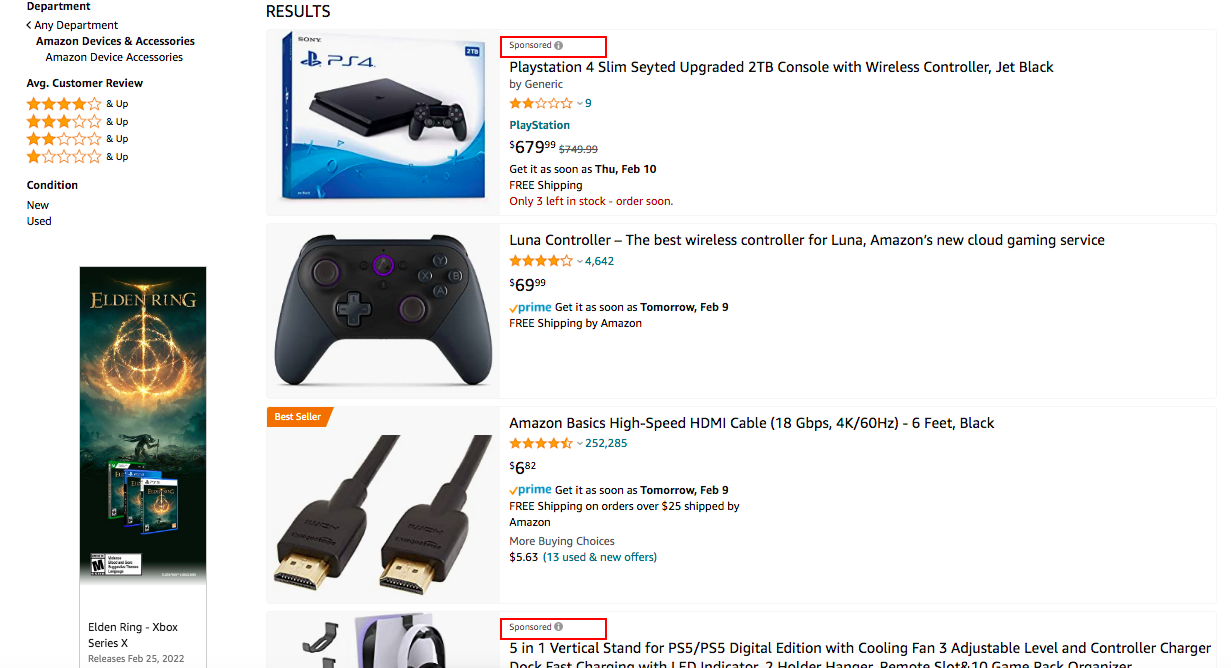Screenshot Description:

The image features a white background, showcasing various Amazon shopping filters and product listings. In the departmental filters section, categories like "Amazon Devices and Accessories" and "Amazon Device Accessories" are present. The customer rating filter offers options ranging from "Four Stars and Up" to "One Star and Up." Additionally, condition filters display options such as "New" and "Used."

Search results include both regular and sponsored listings, identified by a gray circle with a white eye icon. An outlined rectangle highlights a specific product: the PlayStation 4 Slim. The detailed description mentions it as "Upgraded to TV Console with Wireless Controller, Jet Black" and is sold by "Generic." This item has a rating of two stars from nine reviews, priced at $679.99, with the original price of $749.99 crossed out. The availability note states: "Get it as soon as Thursday, Feb 10," and indicates free shipping.

Another featured product is the "Luna Controller," branded as "The Best Wireless Controller for Luna, Amazon's New Cloud Gaming Service." This controller has four stars based on 4,642 reviews and is priced at $69.99. It is available for Prime members and can be delivered as soon as tomorrow, February 9.